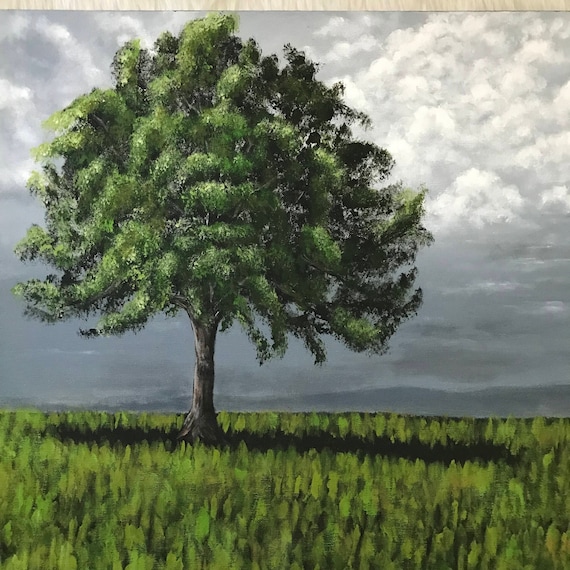This painting on canvas depicts a mature tree standing tall in the middle of a lush green field. The tree's clean trunk extends high, giving way to a vast expanse of thick branches adorned with rich green leaves, forming a shape reminiscent of a smooth-edged triangle or a lollipop. The intricate play of dark and light green foliage creates a striking contrast, especially under the diffused sunlight filtering through a predominantly gray, cloudy sky. The tree casts a distinct shadow below and slightly to the right, adding depth to the scene. In the background, distant gray mountains rise subtly against the darker horizon, blending seamlessly into the various shades of gray in the sky. The serene meadow with its expansive green grass stretches out, leading to the softly glowing mountain range, capturing the tranquil yet moody essence of the landscape.